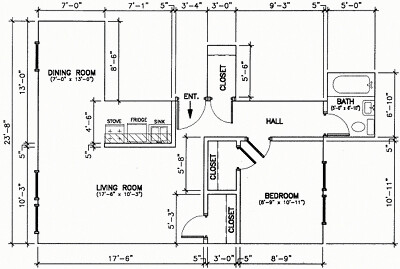This blueprint depicts an aerial view of a single-level floor plan of a house, likely suggesting it could be a second floor but possibly a one-level living area. On the left side, there is a dining room adjacent to a kitchen area labeled with "stove," "fridge," and "sink." Nearby, a living room occupies the bottom-left corner. Centrally located, two closets and a hallway provide access to various parts of the floor. On the right side, the layout includes a bathroom furnished with a tub, toilet, and sink, along with a bedroom. Additionally, there is an unlabeled room next to the bedroom. The blueprint features several entryways and indicates various room dimensions in feet and inches, predominantly around the perimeter, ensuring precise measurements for construction and design.